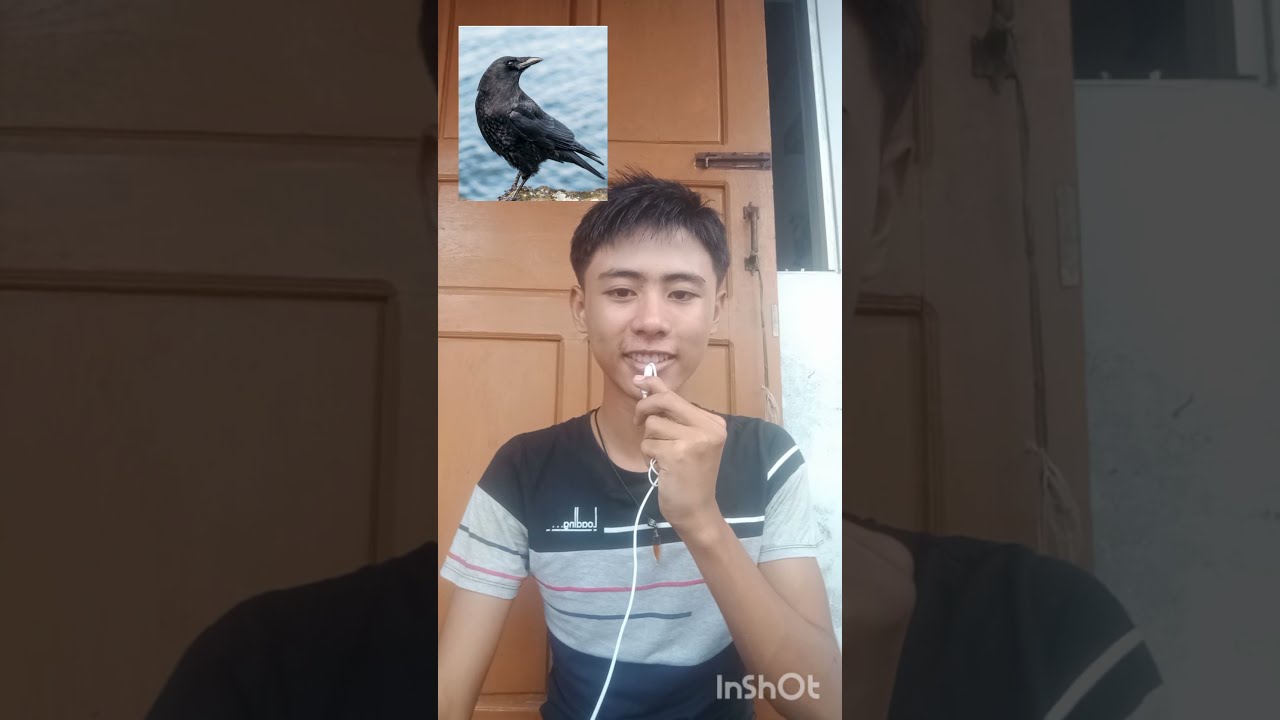The image features a young Asian male with dark hair, wearing a black, gray, and red striped shirt. He is seated in front of a light brown door with a black handle and lock. He is holding a white microphone with a long cord up to his mouth, appearing to speak into it. This central photo is superimposed with two other panels of the same image, one on either side, which capture just the shoulders and are darker and more underexposed. In the top left-hand corner of the central image, above the young man's head, there is a small square containing an image of a black bird standing in or near water. The word "InShot" is also visible at the bottom of the central panel, indicating the use of a photo editing app. The overall effect is a triptych with the main image in sharp focus and the surrounding panels blurred and expanded.